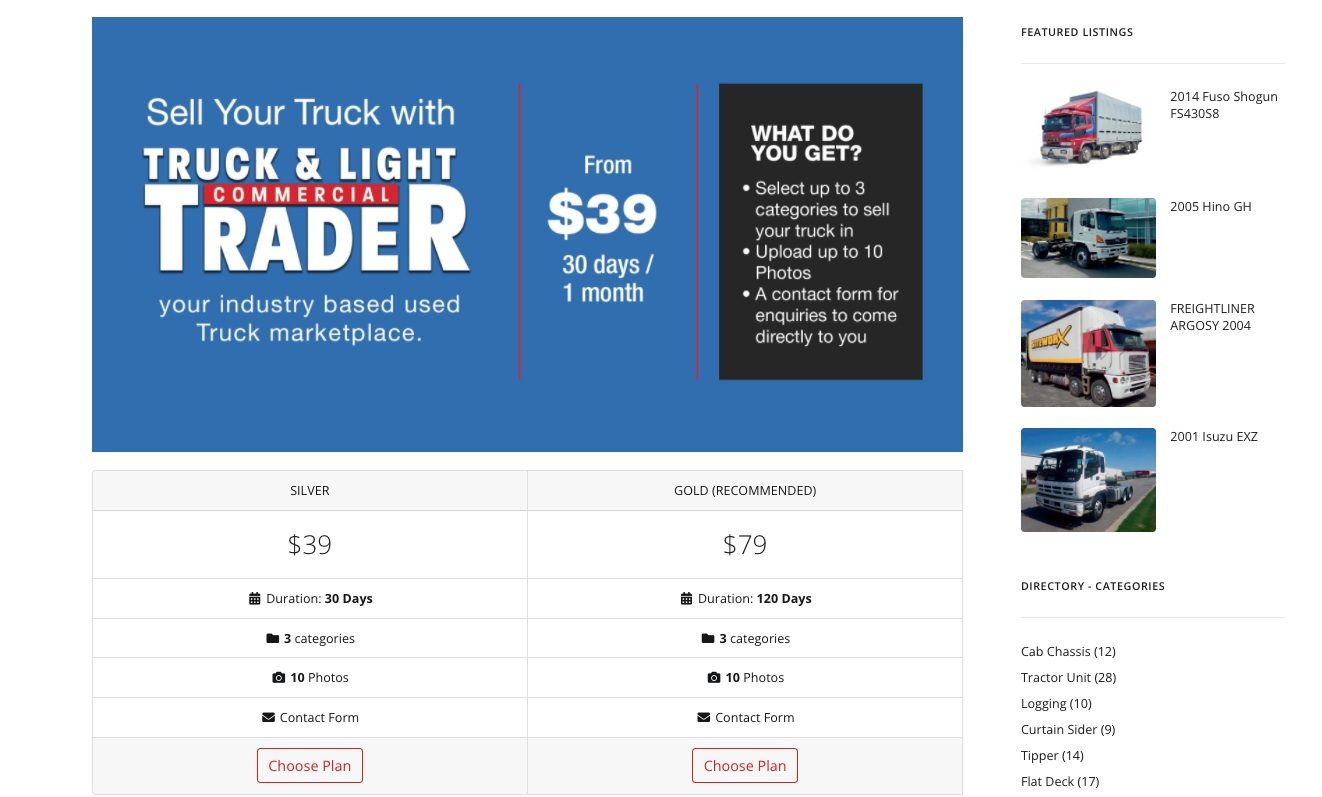The website dedicated to truck sales features a well-structured layout for users. In the upper left corner, a prominent blue square contains the site's description, stating: "Sell your truck with Truck and Light Trader." Below this, a striking red banner reads "Commercial." Directly beneath, a subtext clarifies the site's purpose: "Your industry-based used truck marketplace."

Moving right, the site offers pricing information: "From $39, 30 days to a month." Adjacent to this, a black box outlines user benefits: "What do you get? Select up to three categories to sell your truck in. Upload up to 10 photos. A contact form for inquiries to come directly to you."

To the right, four featured truck listings are displayed, each with corresponding images and descriptions:  
1. 2014 Fuso Shogun - Boxed truck with 12 wheels.  
2. 2005 Hino GH - Model specifics not detailed.  
3. Freightliner Argosy 2004 - Model specifics not detailed.  
4. 2001 Isuzu EXZ - Model specifics not detailed.

In the lower left section, the site details its service plans: the Silver Plan at $39, and the recommended Gold Plan at $79.